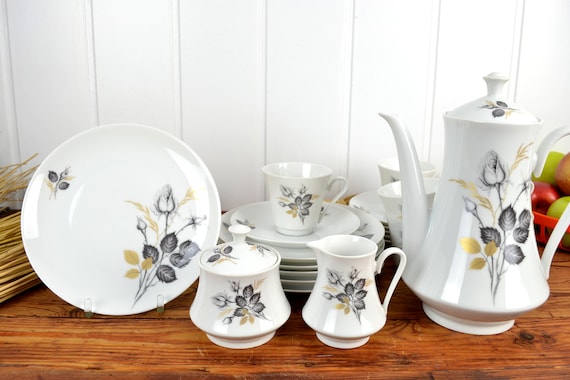The photograph depicts a meticulously arranged china set displayed on a medium-colored wooden table, showcasing its grain with hints of red and yellow hues. The backdrop is a white, segmented wooden wall, painted white, allowing the china set to stand out prominently in the natural, well-lit indoor setting.

Central to the arrangement is a stack of larger plates, topped with a smaller plate on which a tea cup perches precariously. All the china pieces share a harmonious design featuring delicate floral motifs in black, gold, gray, and yellow, predominantly centered around tulips with dark and light green leaves. In the forefront, on the right side, a tall, elegant teapot commands attention with its distinctive arching handle and left-side spout. Beside it, there's a wide, handle-less cup with a lid, likely for sugar or other condiments, adding to the allure of the display.

An additional plate is propped up on the far left, prominently showcasing the tulip design, integrated tastefully with the rest of the set. Complementing the aesthetic arrangement, a basket filled with red and green apples sits to the right, adding a touch of rustic charm and color contrast to the sophisticated display. The overall composition not only highlights the intricate details and cohesive design of the china set but also evokes a sense of traditional elegance and curated simplicity.